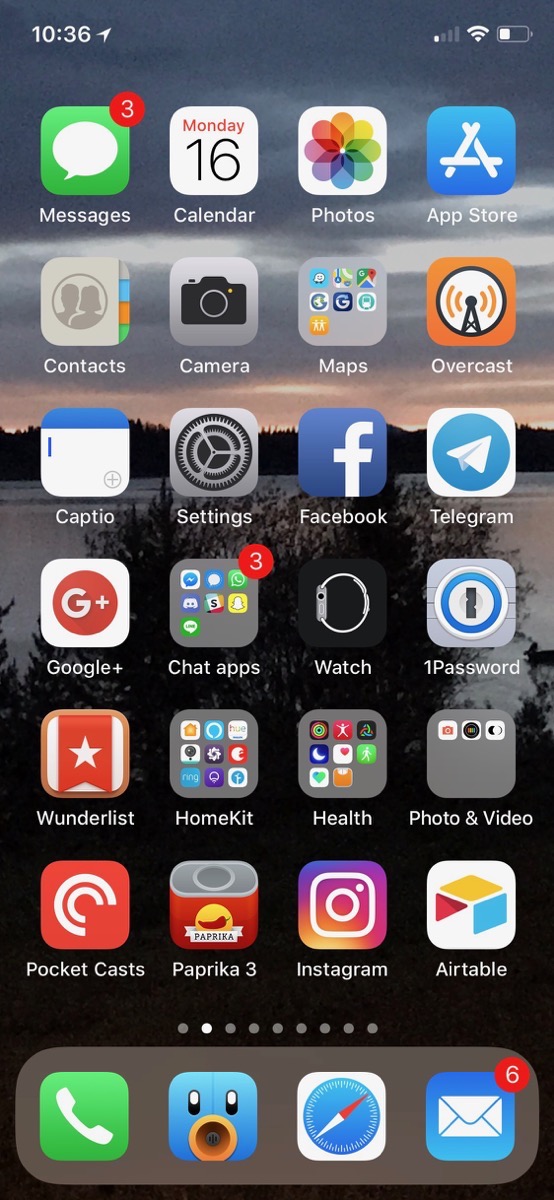The image showcases the home screen of a cell phone featuring a dark, stormy, cloudy sky wallpaper with a tree line overlooking a lake and a bush in the foreground. The status bar at the top displays the time as 10:36 in the upper left corner, a weak data signal (1 of 4 bars), full Wi-Fi signal (3 of 3 bars), and a one-third filled battery icon in the upper right corner.

The main screen is dotted with various app icons. Notably, the Messages app has a notification badge with the number 3. The other icons visible include: Calendar showing Monday the 16th, Photos, App Store, Contacts, Camera, Maps, Overcast, Cappsio, Settings, Facebook, Telegram, and Google Plus. There’s a folder labeled "Chat Apps" also displaying a notification badge with the number 3.

Additionally, there are icons for Watch, 1Password, Wunderlist, HomeKit, Health, Photo & Video, Pocket Cast, Paprika 3, Instagram, and Airtable. At the bottom dock, there are four icons: a Phone, a blue character with a surprised expression, a Compass, and a Mail app with a red notification badge showing the number 6.